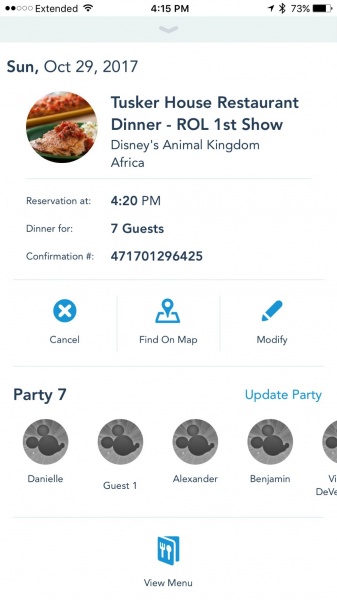In this image, we see a structured interface on a white background. At the very top, there are five small circles, with two highlighted in black. The status shows "extended for 15 p.m." and indicates a battery level of 73%. Below, there's a blue rectangle featuring a down arrow icon.

Next, a white box displays the date "Sunday, October 29th, 2017," along with a small circular icon containing an image. This section includes text that states "Tusker House Restaurant, Dinner, ROL, First Show, Disney's Animal Kingdom, Africa."

Following this, a horizontal blue line highlights the reservation details: "Reservation at 4:20 p.m., Dinner for seven guests," along with the confirmation number "471701296425." Under this line, three interactive buttons are displayed— "Cancel," "Find on Map," and "Modify."

Another horizontal line separates this section from the party details. Here, names in circular icons are presented, listing "Danielle, Guest One, Alexander, Benjamin," and partially visible additional names.

At the very bottom, there is another option labeled "View Menu," accompanied by an icon illustrating a fork and spoon.